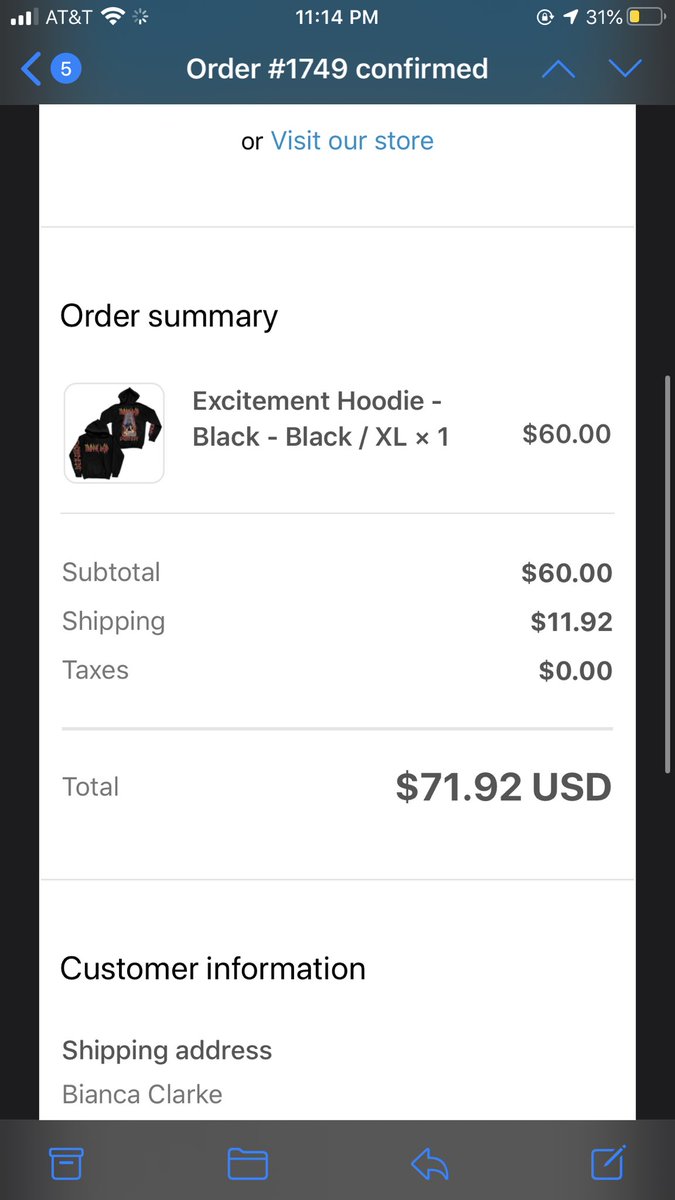This image is a detailed screenshot of an order confirmation for a sweatshirt on a smartphone. The phone is connected to AT&T, showing three to four signal bars and full Wi-Fi reception. The time on the device is 11:14 PM, and the battery is at 31%. At the top of the screen, there is an animation of a spinning loading icon.

The main content of the screen includes a blue back arrow and a blue circle with a white number "5" inside it. Below this, the text "Order Number 1749 Confirmed" is prominently displayed, accompanied by up and down arrows on the right side and a pop-up message offering to "Visit Our Store." The background of the screen is white with text segments on it.

An order summary is provided beneath a small thumbnail of a black over black XL hoodie, labeled as the "Excitement Hoodie." The order details specify one item costing $60, with a subtotal of $60, shipping fees of $11.92, zero taxes, and a total amount of $71.92, which is highlighted in larger text.

Further down, there is a section titled "Customer Information" showing the shipping address tied to the name Bianca Clark. The screen ends with a gray bar featuring four electric blue icons: a box, a manila folder, a back arrow, and a pen on a tablet.

Additionally, there's a light gray scroll bar on the right side, and a faint glimpse of the device's background wallpaper is visible.